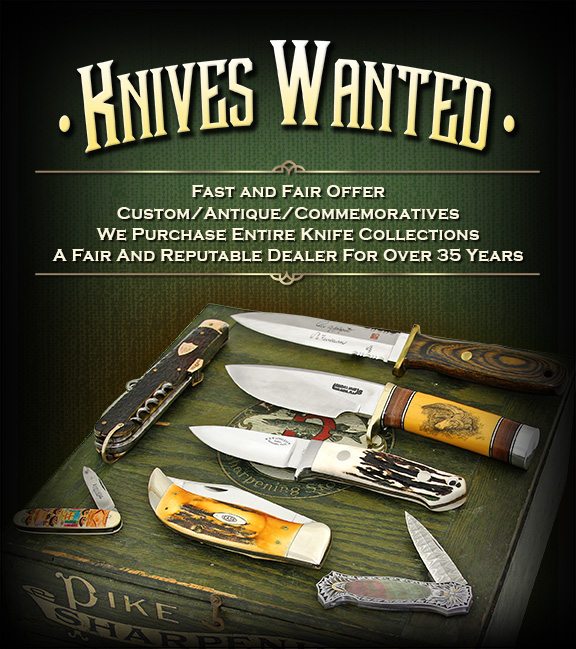This rectangular advertisement, approximately five inches high by four inches wide, features a green backdrop with a darkened vignette around the corners and top edge. Dominating the top section is the bold title "Knives Wanted," with a gradient color shift from white at the top to light yellow at the bottom, flanked by bullet points. Below this, white text on horizontal lines reads: "Fast and Fair Offer, Custom, Antique, Commemoratives. We purchase entire knife collections. A Fair and Reputable Dealer for over 35 years."

The lower half of the image showcases an assortment of knives resting on an old wooden box marked "Pike Sharpeners." Visible are various types of knives, including hunting knives, carving knives, and at least one Swiss Army knife. The handles show signs of wear, with some featuring vibrant yellow or colorful designs, while others are more understated. This poster serves as an advertisement for a knife dealer, highlighting their long-standing reputation and fair purchasing practices.